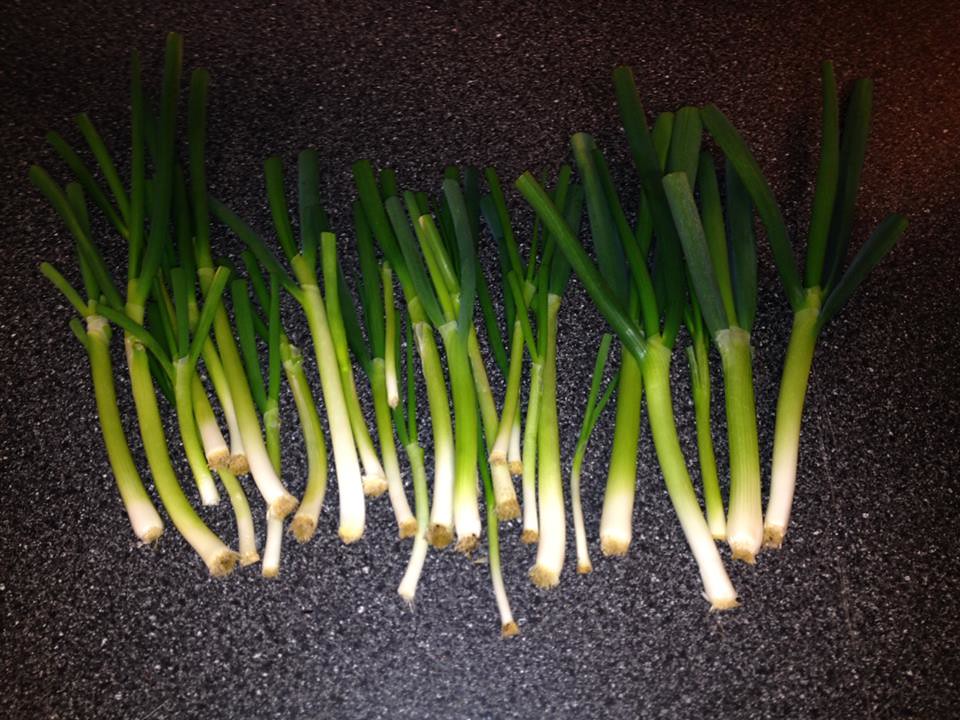The image features approximately 28 green onions arranged horizontally across a rough, black, pavement-like background, speckled with white dots. Each green onion showcases a vibrant gradient, starting with deep hunter green stems at the top, transitioning to a lighter pea green towards the middle, and finally ending in a white bulb at the base. Most onions still have small, brownish roots attached, indicative of their recent harvest. The green onions, some longer and thicker than others, are uniformly aligned with the green tops towards the top of the image and the white bases at the bottom, creating a visually striking and orderly display.